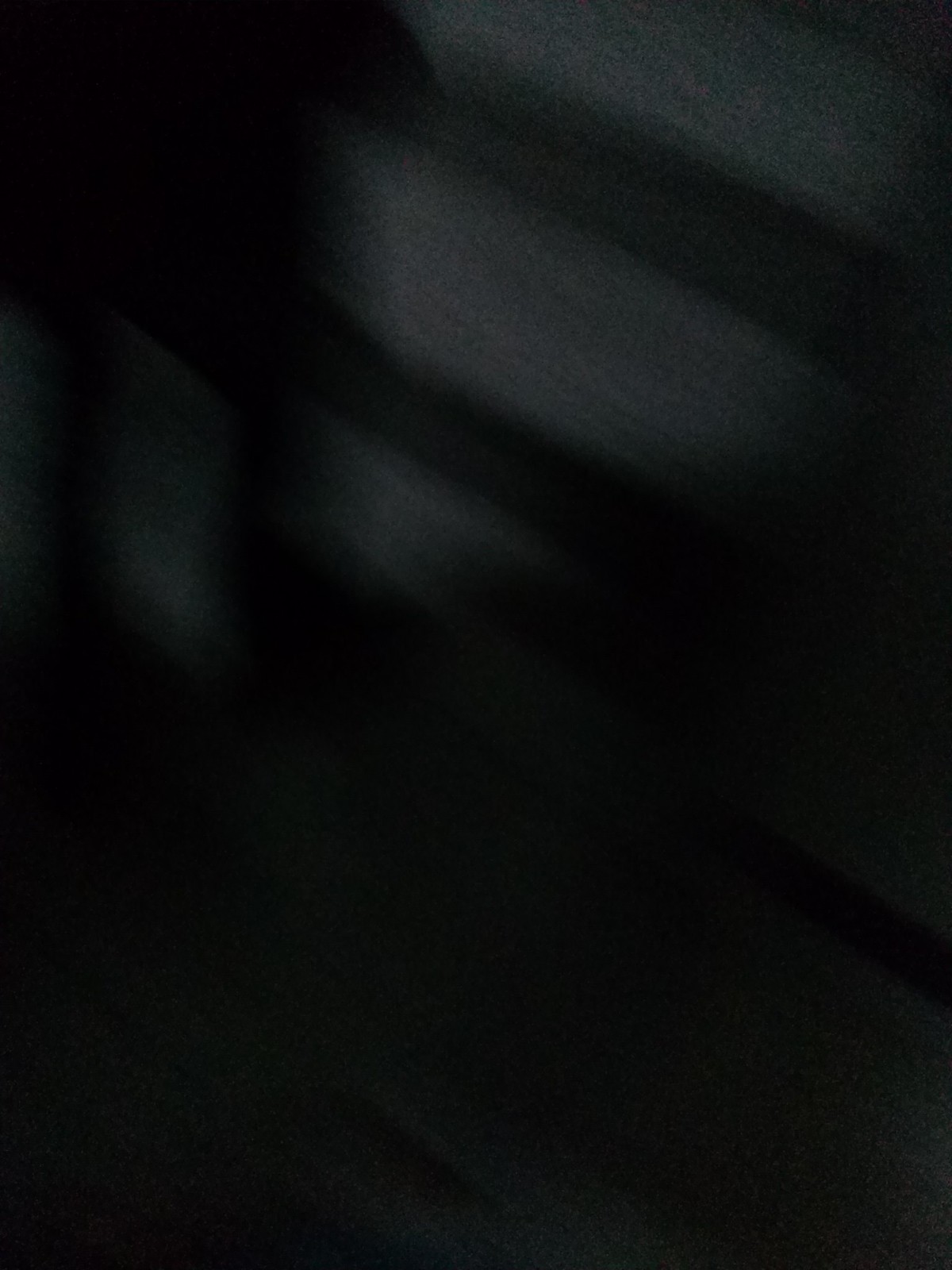**Caption:**

A predominantly dark image with an almost entirely black background, devoid of any discernible objects. Near the top half of the image, there are three distinct white streaks crossing the frame. The uppermost streak spans about half the width of the image. Below it, slightly angled, is a second streak that is almost as long. Further down, a significantly smaller streak is visible, accompanied by another tiny streak to its left. These streaks are highlighted with a subtle black outline, adding contrast to the otherwise stark and minimalistic image.